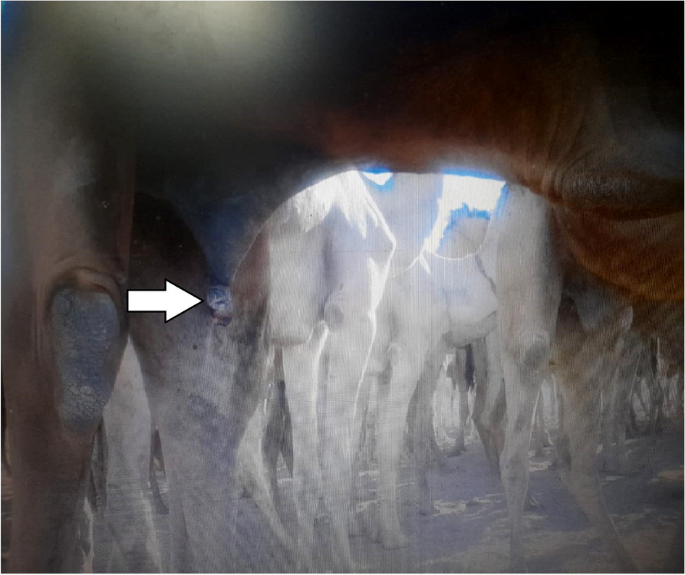The image depicts the underside of a brown horse, viewed from beneath, with a distinct white arrow pointing at a small bump on the horse's inner leg, possibly indicating an area of concern or injury. The scene is slightly blurry and uneven in focus, making details less clear. Surrounding the brown horse are numerous white or beige horses, with the view capturing mostly their legs and torsos. These horses appear tall, with long legs and their lower limbs showing white hooves. The background blends a white and grayish ground with patches of bright sky visible through the horse's middle section and between the heads of the other horses, suggesting it is daytime.